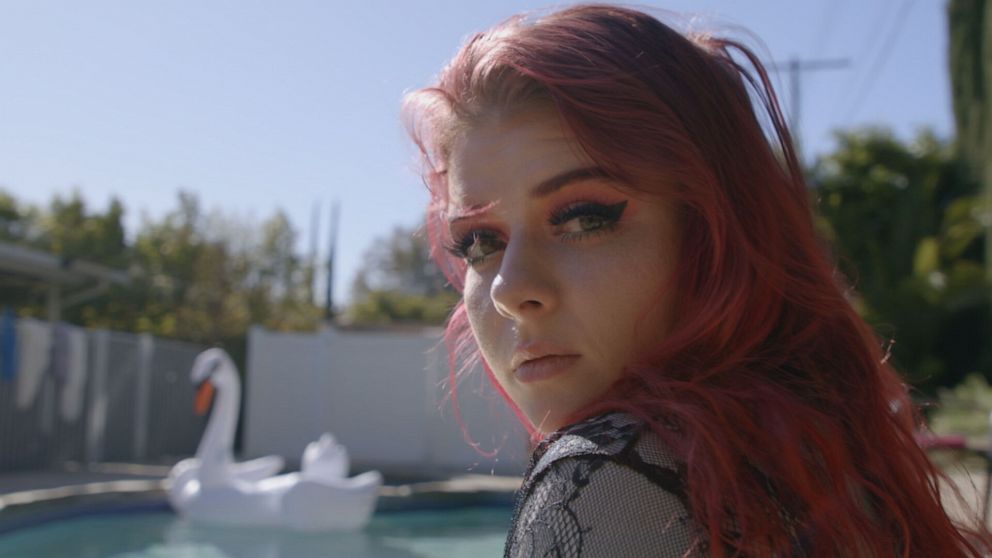The photograph features a young white woman with long, dyed red hair, wearing a sheer black and gray lace top. She has pale skin and is adorned with green and red eyeshadow, giving her a serious expression. The close-up shows her looking back over her left shoulder toward the camera. She is seated near a swimming pool in what appears to be a backyard surrounded by gray stone walls. The pool prominently features an inflatable white swan float with an orange beak. Beyond the pool, there is fencing and a backdrop of tall green trees under a bright blue sky, indicating a clear, sunny day. The image captures a well-lit, outdoor setting with no other people present.